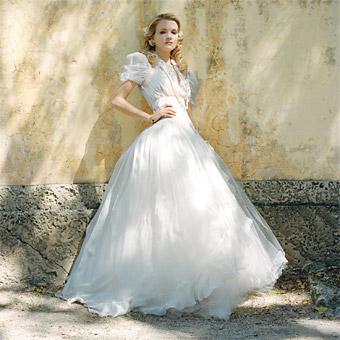The image features a Caucasian woman with blonde hair, styled long and loose, posing in a white, fluffy wedding dress. The dress is characterized by its puffy shoulders, which are short-sleeved, and extends down, obscuring her feet with its voluminous tulle fabric. She stands confidently, looking directly at the camera, with one hand on her hip and her elbow bent outward. Notably, she is wearing a gold watch on her wrist. The background reveals a tan, cream-colored wall that appears pale due to the sun's reflection, contrasted by a darker gray stone along the bottom. The ground beneath her is composed of crushed stone, adding texture to the scene.